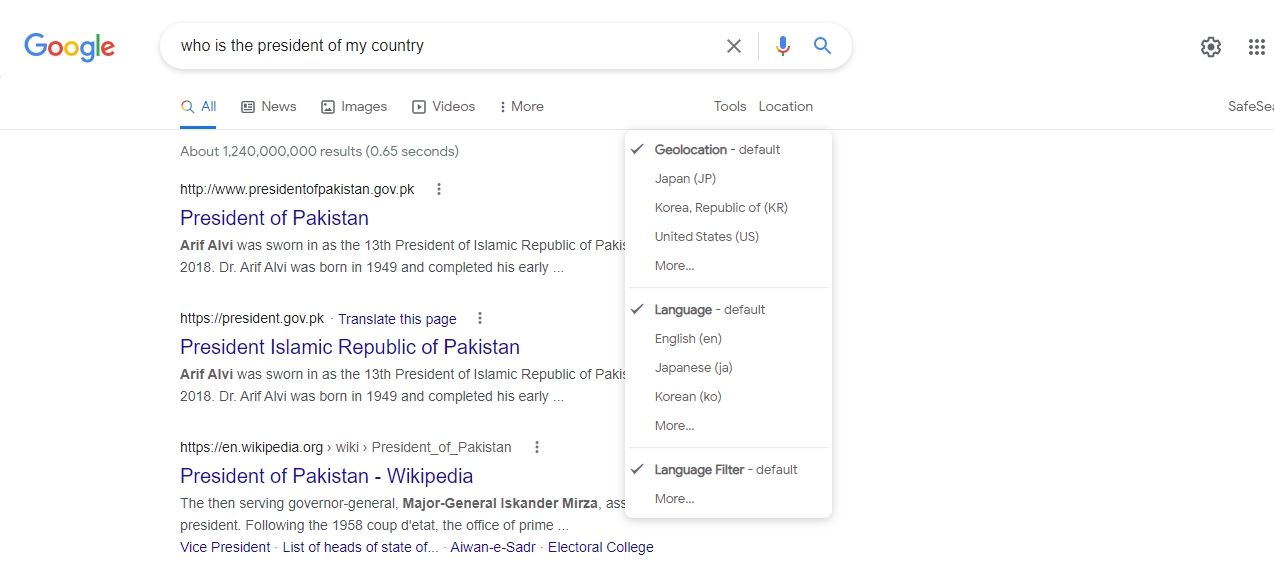This is a detailed screenshot of a Google search results page, showcasing various elements of a typical query interface. In the upper left corner, the iconic Google logo is prominently displayed, with its letters colored blue, red, yellow, blue again, green, and red in sequence. Adjacent to the logo is a long, rectangular search bar with rounded edges, containing a user-entered query, "Who is the president of my country?" in black text.

To the right of the search bar, three distinct icons are visible: a dark gray 'X' for clearing the query, a blue and red microphone symbolizing the speech-to-text feature, and a blue magnifying glass indicating the search function.

Beneath the search bar, the page indicates approximately 1.24 billion search results achieved in 0.65 seconds. The displayed search results highlight information related to the president of Pakistan. The titles and snippets suggest links to the official role, including a page from Wikipedia dedicated to the President of the Islamic Republic of Pakistan.

The background of the page is white, with navigation options at the top, including tabs labeled "All," "News," "Images," "Videos," and "More," allowing users to filter their search results based on content type. This screenshot captures the essence of a Google search page layout and user interface details efficiently.